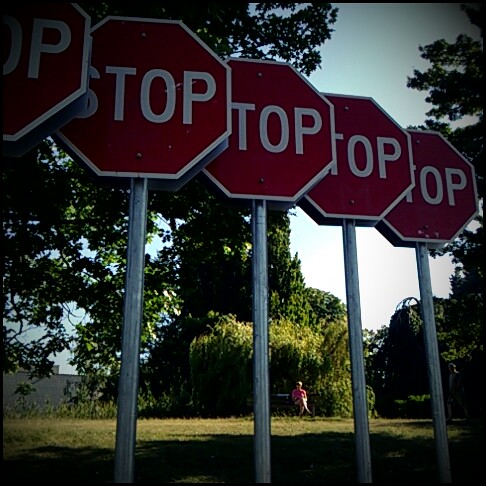This is a color photograph, possibly digital and square in format, showcasing an intriguing arrangement of five stop signs aligned closely together, their dark red, well-preserved lettering interweaved and partially obscured from a perspective looking upward. The image has darkened edges, creating a vignette effect that draws attention to the central composition. The stop signs, mounted on typical metallic poles, appear almost stacked like plate armor or scales, suggesting these might be set against a park-like scene or perhaps awaiting installation. In the background, amidst a mix of overgrown trees and bushes, a figure wearing a pink (or possibly red appearing in the light) shirt and shorts can be seen sitting on a park bench. They sit relaxed in a patch of sunlight breaking through the otherwise shady environs cast by tall trees. The surrounding lawn is a blend of green and brown, indicating a space that is maintained but not meticulously manicured. The scene evokes a quiet, slightly surreal environment that mixes elements of everyday suburban life with an unusual and thought-provoking display.